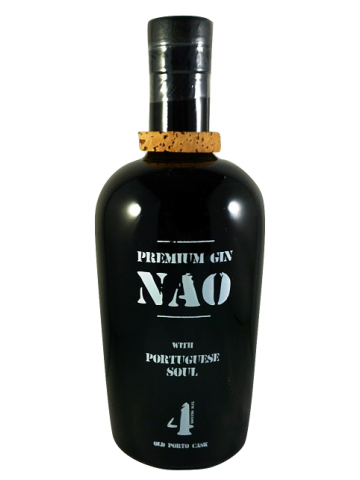The image depicts a sleek, black bottle of gin, strikingly contrasted against an all-white background. The bottle features a distinctive black cap covered by a plastic seal, which includes an orange ring at its base. Surrounding the neck is a brown cork material that adds a rustic touch. The bottle is adorned with white text, starting with the words "Premium Gin" prominently displayed below a horizontal line. Further down, the bold letters N-A-O are followed by "With Portuguese Soul" and a large number "4" near the bottom. Though the very bottom text is partially obscured, it includes additional, smaller white letters. The overall bottle has a shiny finish, highlighted by reflections of white light, indicating that the photograph was likely taken indoors.